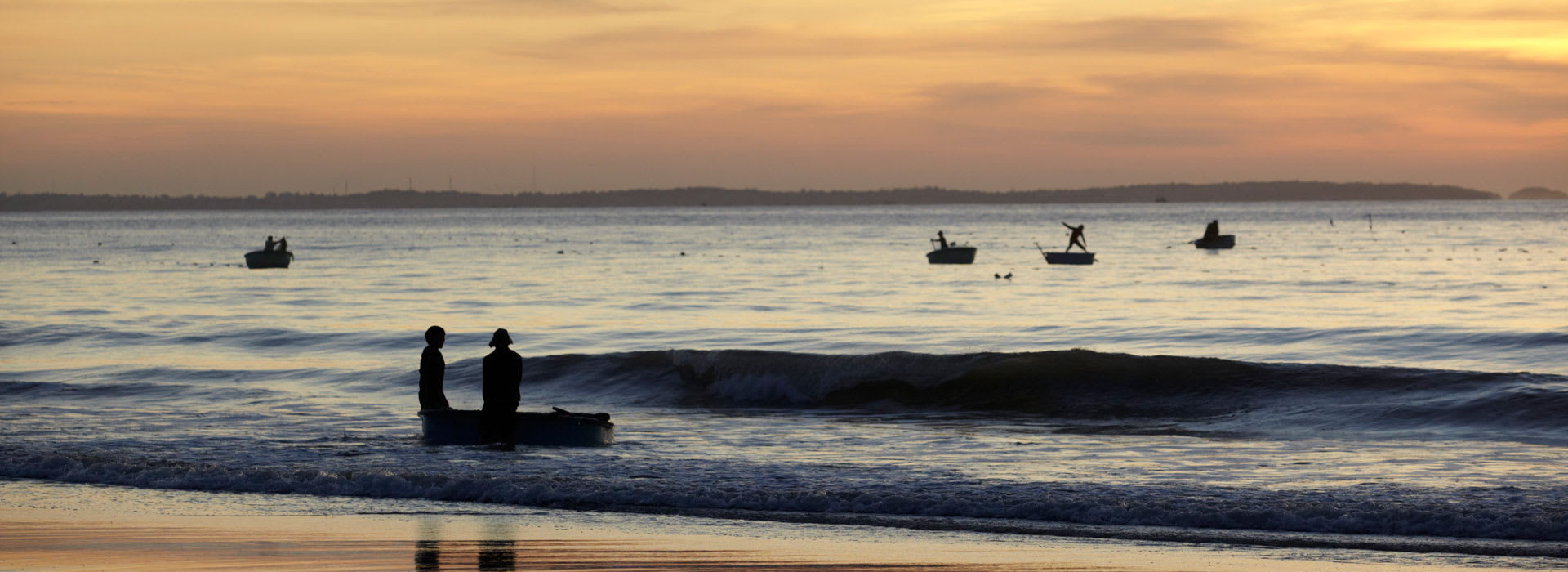This photograph captures a serene beach scene at sunset, facing west. The sky is painted in rich hues of orange, pink, and yellow, with a few clouds scattered across it. The sun's light reflects off the almost white water near the horizon, creating a luminous effect. In the background, there's a dark strip of low-lying land or mountains dividing the sky and the water.

In the middle of the image, the calm ocean is dotted with five small vessels, resembling canoes or fishing boats. The closest boat to the shore has two people standing beside it, appearing almost like silhouettes as they possibly push the boat into the water. In the distance, there are four more boats, each occupied by one or two shadowy figures, floating serenely. The water is relatively calm, with gentle waves lapping onto the sandy shore at the bottom of the photograph.

The combination of the silhouetted figures, the calm waves, and the warm, colorful sky creates a tranquil and picturesque coastline moment.